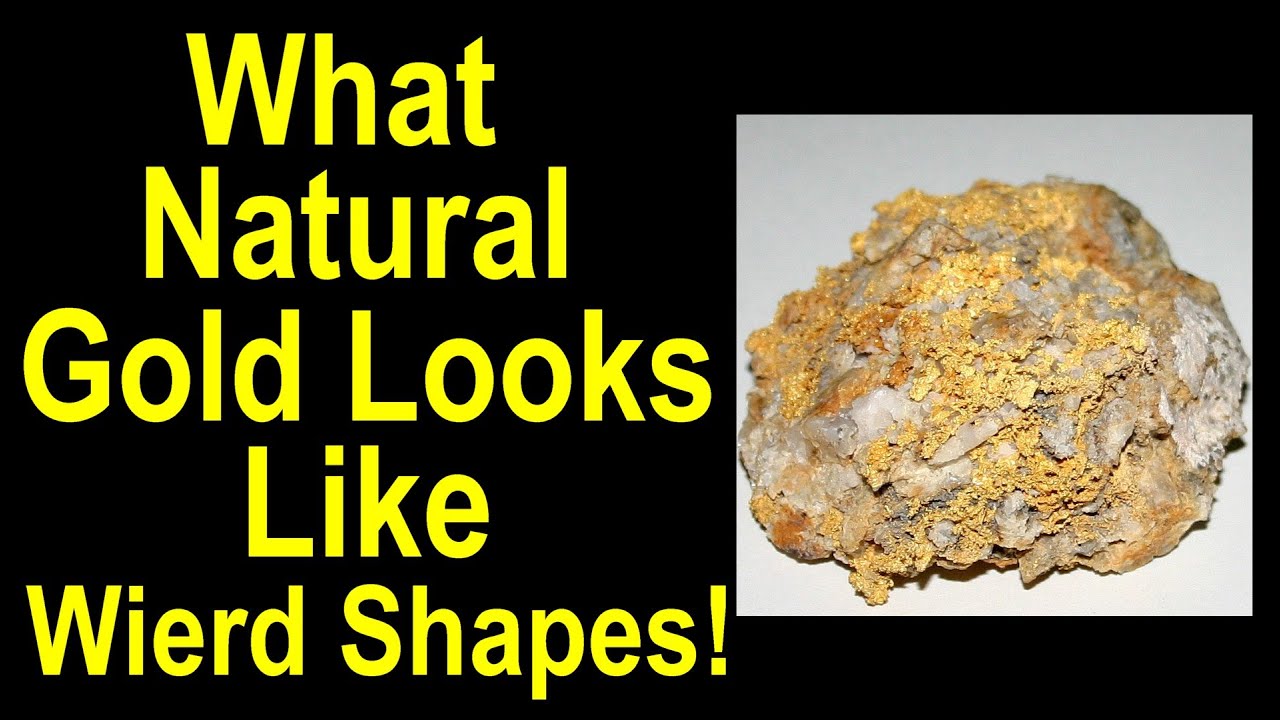This image features a striking display set against a black background. On the left-hand side, bold yellow text reads: "What natural gold looks like - weird shapes!" To the right, there is an intriguing rock specimen prominently displayed. The rock itself is mainly tan in color, interspersed with black specks, transitioning into a goldish hue in the middle. A quartz segment, situated at the left tip, is white and somewhat translucent. Throughout the rock, gold flakes are scattered, appearing almost as if they are adhered to the surface like moss. The backdrop behind the rock is an understated light gray-blue, providing contrast to highlight the rock's intricate details and the unique formation of the gold, which seems to cling in various shapes around the quartz.